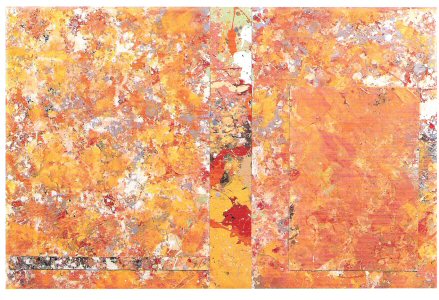The image is a very modern and abstract painting characterized by its splotchy and seemingly random application of colors. Dominantly featuring shades of yellow, orange, and a brownish-red mixed with white and black speckles, the painting is bereft of identifiable objects, giving it an experimental, almost Jackson Pollock-esque quality. Central to the composition are two large vertical rectangles positioned in the middle, flanked by smaller, irregular blocks on either side. The background appears predominantly white, with the colors giving an impression akin to fall leaves from a distance. The lower section of the painting includes two more long horizontal rectangles, separated by the central vertical rectangles. The colors are intricately blended, almost marbled in appearance, which adds to the complexity and layered texture of the piece. The left side shows a more defined roughness, while the right side blends the colors more smoothly. Overall, this rectangular painting contains no signature and conveys a highly abstract, modern artistic style.